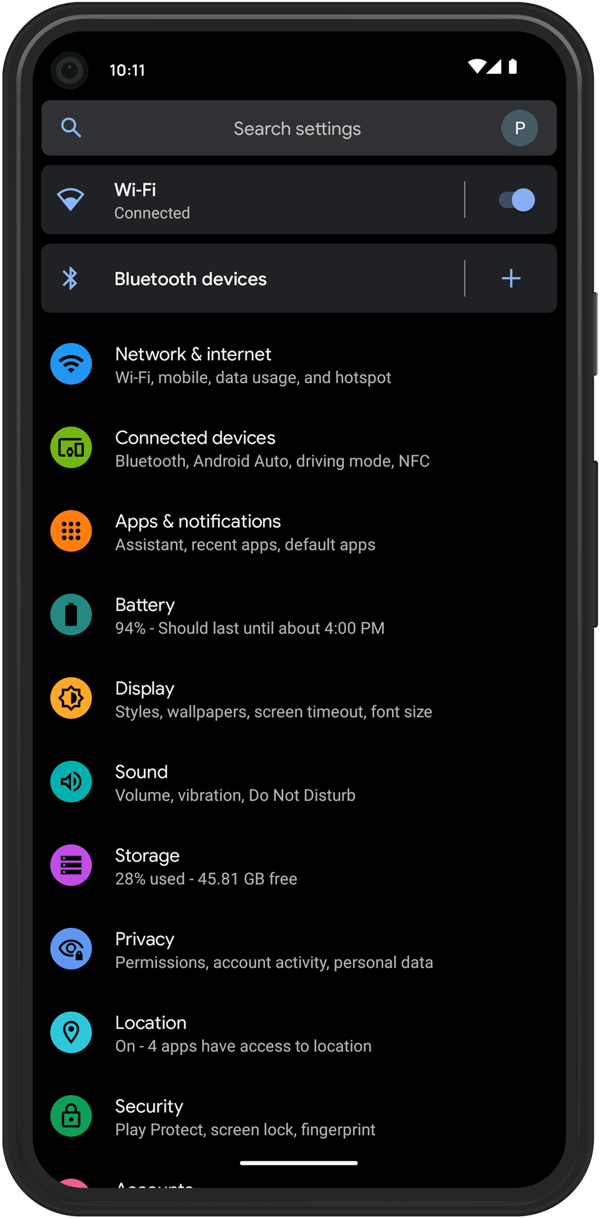The image showcases a detailed view of a cell phone’s settings menu displayed on a black background. In the top-left corner, the time is indicated as 10:11. The top-right corner features three icons: Wi-Fi, connection status, and battery percentage. Directly beneath, a rectangular search bar labeled "Search settings" is positioned, flanked by a magnifying glass icon on the left and a circular "P" icon on the right.

Centered beneath the search bar, the Wi-Fi setting is displayed as connected and toggled on. Next in line is the Bluetooth devices section. Below this are various settings categories listed from top to bottom, each accompanied by a uniquely colored circle with the category's icon. The colors of the circles are, in order: blue, green, orange, blue, light orange, light blue, light purple, blue, light blue again, green, and a small visible portion of a pink circle at the bottom left corner.

To the right of each circle, the category names are clearly written in white text. They are listed as: Network and Internet, Connected Devices, Apps and Notifications, Battery, Display, Sound, Storage, Privacy, Location, Security, with the final category obscured and unreadable. Examples of each category’s contents are written in smaller text beneath the category names. Notably, the top three options feature light gray rectangular backgrounds, contrasting against the predominantly black background of the screen.